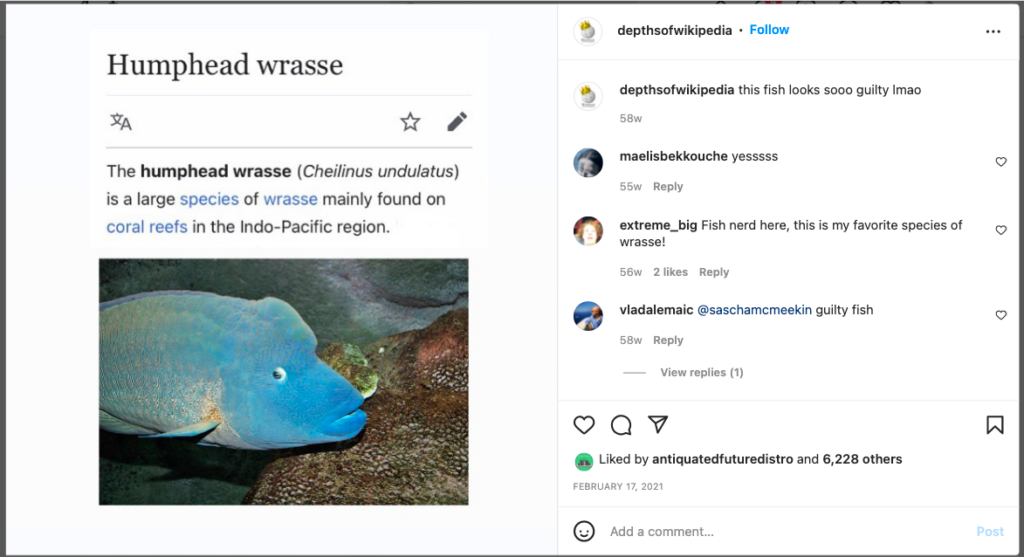This image is a partial screenshot showcasing both a Wikipedia entry on the left and a social media conversation on the right. The Wikipedia page features the humphead wrasse (Cheilinus undulatus), a large fish species predominantly found on coral reefs in the Indo-Pacific region. Just under the text is a photograph of a vivid blue humphead wrasse, orientated to the right and looking at the camera with its eye humorously rolled to the side, which gives the fish a slightly comical expression.

To the right of the Wikipedia entry is a fragment of a social media conversation. The discussion is titled "Depths of Wikipedia," where users comment on the fish's appearance. One user remarks, "This fish looks so guilty. LMAO," followed by "Maelis Bekkouche" affirming "Yes." Another user, "extreme_big_fish_nerd_here," shares their admiration, stating, "This is my favorite species of wrasse." Another comment by "Vladalemai" at "Saschamcmeekin" humorously labels the fish as "Guilty fish." The post is liked by users "Antiquated," "FutureDistro," and 6,228 others. The social media interaction is timestamped February 17, 2021.